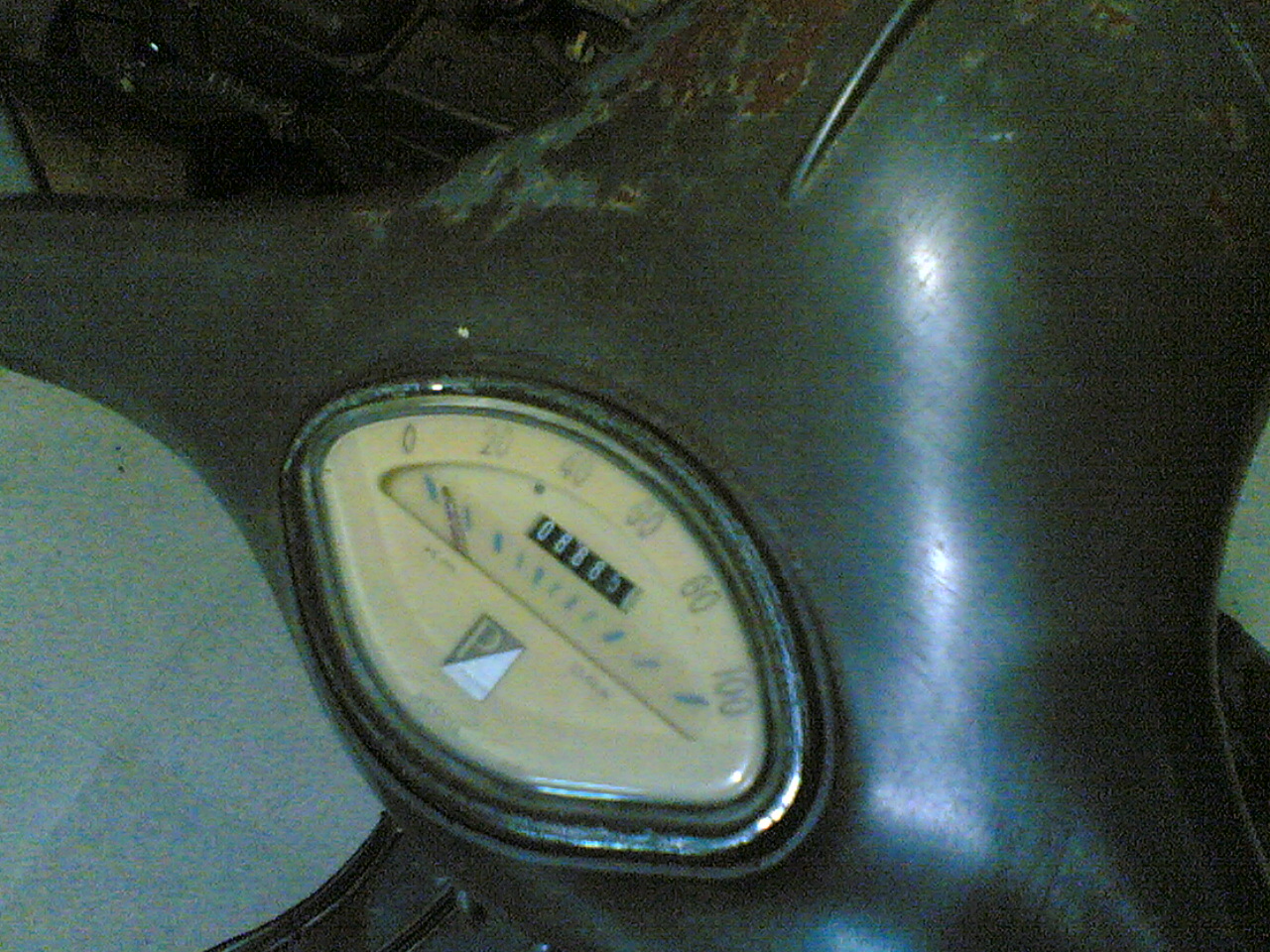A dimly lit photograph captures the close-up of an aged motorcycle or scooter odometer, with its focal point being the vintage-styled speedometer. The odometer, set against a cream-colored background, prominently displays even numbers 0, 20, 40, 60, 80, and 100, encircling a small central dial. This central mile counter, though slightly blurred, indicates a reading of 8,885 miles. The speedometer, housed in an oval-shaped frame, shows signs of wear and age, with noticeable rust and patina at the top, contributing to its vintage allure. The brand of the vehicle is indiscernible due to the shadowy ambiance. In the top left corner of the image, an indistinct object looms in the darkness. The scene is further detailed by the flooring, which resembles garage-style gray tiles rather than household tiles, suggesting the vehicle is parked in a garage environment. The overall atmosphere exudes nostalgia and the rich history of the weathered two-wheeler.